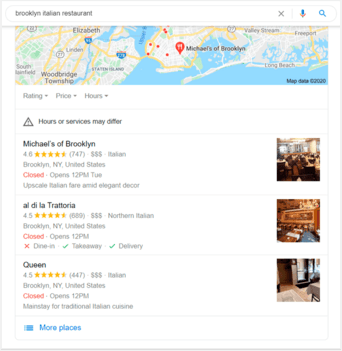This screenshot from MapQuest displays a search for Italian restaurants in Brooklyn. The search term "Brooklyn Italian restaurants" is clearly visible in the search bar at the top of the page. Below the search bar, a map is featured with various filter options for rating, price, and hours, allowing users to organize their search results. A caution icon with a triangle and exclamation point warns that hours or services may differ. 

The first search result is Michael's of Brooklyn, boasting a 4.6 rating from 747 reviews. This restaurant, which is identified by its three dollar signs as a more expensive option, offers upscale Italian fare amid elegant decor. It is currently closed but will open at 12 p.m. on Tuesday.

The second result is Aldia La Trattoria, which has a 4.5 rating from 689 reviews and serves Northern Italian cuisine. 

The third result is Queen, holding a 4.5 rating from 447 reviews, also specializing in Italian food. All three restaurants are located in Brooklyn, New York, United States.